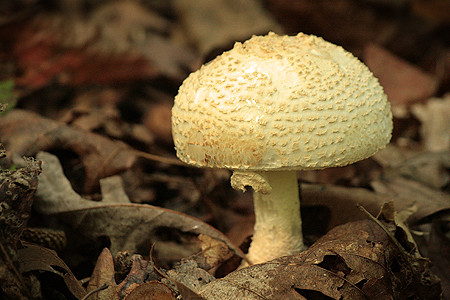In this close-up image, we see a detailed view of a yellowish-beige mushroom emerging from the forest floor. The mushroom boasts a thick, ribbed stem that supports a round, speckled cap, adorned with rough indentations that give it a textured appearance. Surrounding the mushroom are layers of dry, decaying leaves in shades of gray, brown, dark green, and hints of red, creating a stark contrast against the vibrant fungus. The leaves appear abundant and crinkly, suggesting a rich, decomposing leaf litter on the ground. A notable feature of the mushroom is a growth hanging underneath its cap, adding to its unique structure. The overall scene captures the resilience of the mushroom thriving amidst the muted hues of the forest debris.